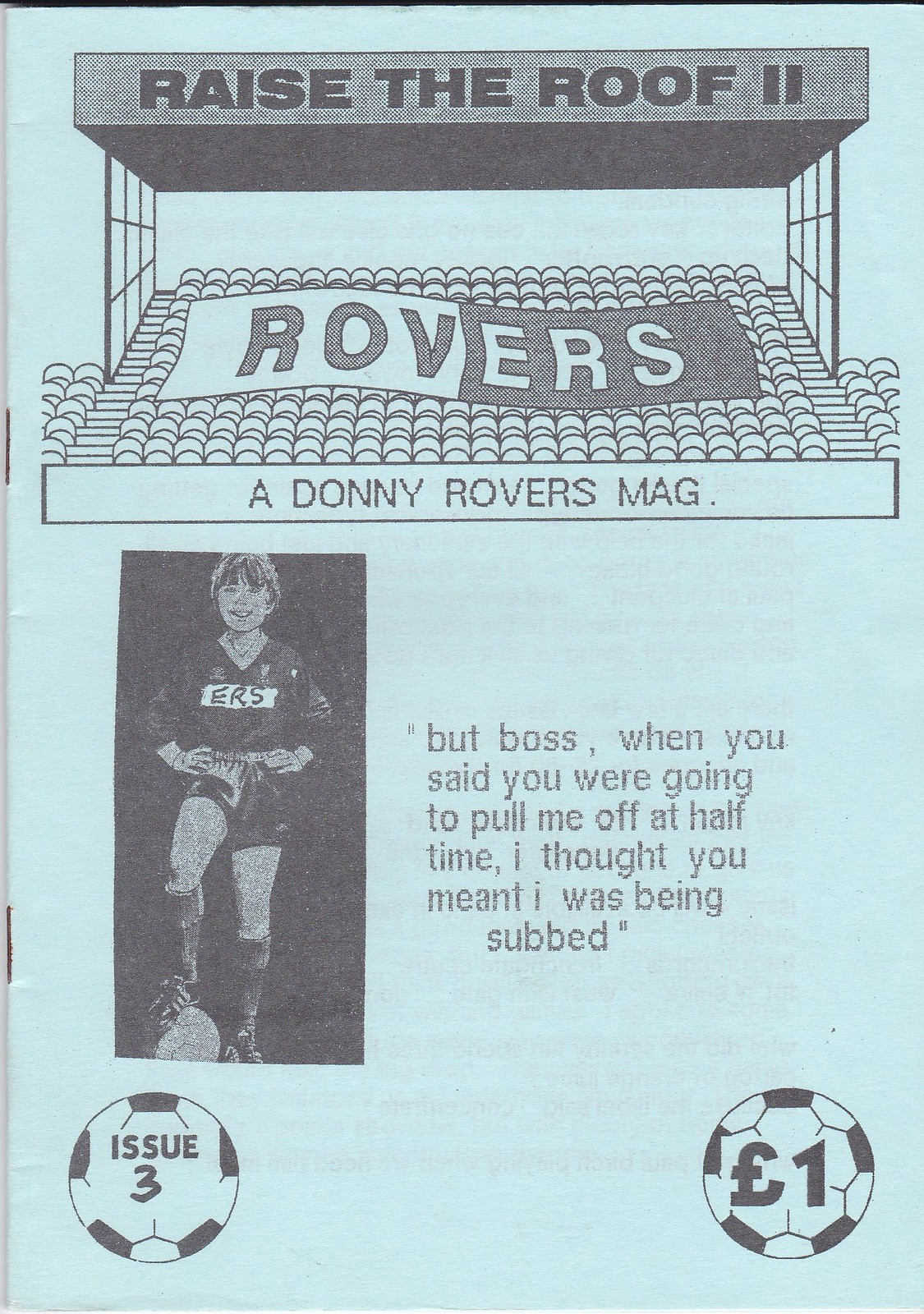The magazine cover features a light blue background with the title "Rovers" prominently displayed at the top, alongside the phrase "Raise the Roof" and a graphic of a stadium with a flag across the seats. Below this, it reads "A Donny Rovers Mag" within a box. On the left side of the cover, there is a black-and-white image of a young soccer player, possibly a boy or girl, dressed in their uniform with the letters "E.R.S." printed on the jersey. The player has a soccer ball under their foot. Beside the image, there is a humorous quote: "But boss, when you said you were going to pull me off at halftime, I thought you meant I was being subbed." In the bottom corners of the cover, the issue number "Issue 3" and the price "1 Pound" are displayed, marked with small soccer ball icons.